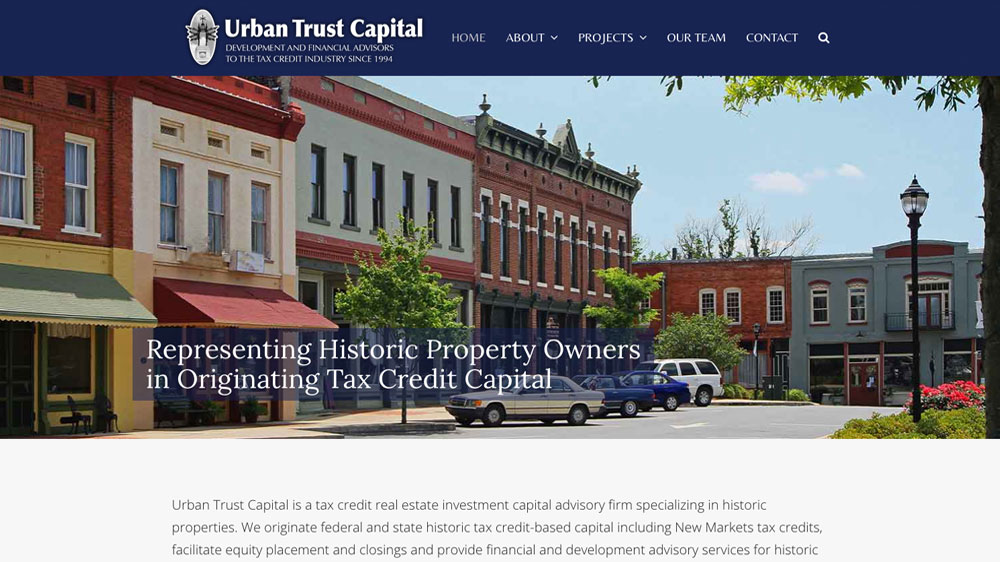In the image, the top section of the webpage showcases a navy background with white text that reads, "Urban Trust Capital, Development and Financial Advisor to the Tax Credit Industry since 1994." Positioned in the top right are navigation tabs labeled Home, About, Projects, Our Team, Contact, and a Search icon.

The central portion of the page features an image of various buildings, accompanied by a caption: "Representing Historic Property Owners and Originating Tax Credit Capital." Below this, a detailed description of Urban Trust Capital is set against a grey background with grey and black text. The text describes the firm as a tax credit, real estate, investment, and capital advisory firm specializing in historic properties. Specified services include originating federal estate and historic tax credit-based capital, including new market tax credits, equity placement facilitation, closing services, and financial development advisory services for historic properties.

The building image prominently displayed in the center consists of structures with diverse architectural styles and colors. These include grey and brick-walled buildings in shades of brown and dark brown. Four cars are visible in the background—one brown, two blue, and one white—complemented by green-leaved trees. The backdrop features a blue sky with scattered light clouds, and the bottom right corner of the image is adorned with vibrant red flowers.